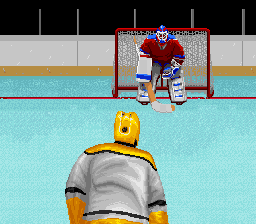This image is a detailed, color rendering, possibly AI-generated or drawn, showing an ice hockey scene on a rink with a very pale aqua blue surface. The background of the rink features a cream wall with narrow white pillars, black at the top, and a yellow line at the bottom. Along the boards, there is a white border with a yellow-colored base and clear glass, set against a dark black background. In the center and just off-center to the back, a hockey goalie stands in front of a red net. The goalie is dressed in a maroon top, wearing a blue helmet and white pads with navy blue accents. He holds a hockey stick in his right hand and is poised in a defensive stance. Approaching him from the front bottom center of the image is another hockey player in a white uniform with yellow stripes and black trim. This player also wears a yellow helmet and is skating toward the net, seemingly ready to challenge the goalie. The overall composition and vivid details suggest this could be from a video game or a digitally created artwork rather than a real-life photograph.